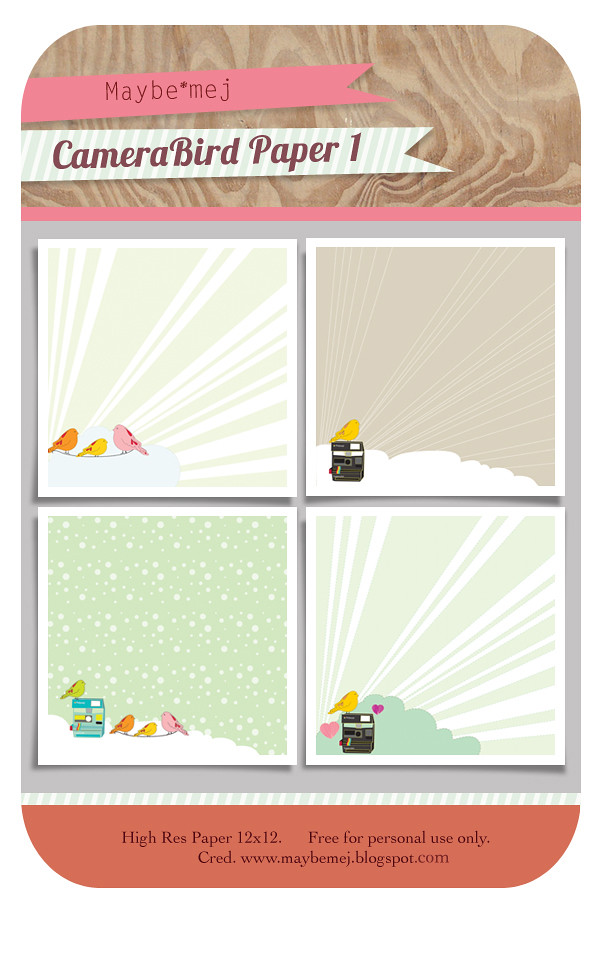This image, likely used as marketing material for a company, features a collection of artistically designed squares each showcasing various bird motifs atop cameras. The header at the top, set against a wood grain background, reads "Maybe Medge, Camera Bird Paper One." Beneath this header are four equally sized squares arranged in a grid pattern, each presenting a unique bird-themed stationery design. In the top left square, an orange, yellow, and pink bird stand out against their background. The top right square features a single yellow bird perched on a Polaroid camera. The bottom right square displays another yellow bird on a camera, surrounded by a whimsical pink heart and purple heart. The bottom left square uniquely showcases four birds—green, orange, yellow, and pink—standing on what appears to be a camera, against a backdrop of white, green, or brown stripes with sun rays. At the bottom of the image, text reads "High Res Paper 12x12, free for personal use only," along with a website for further details.